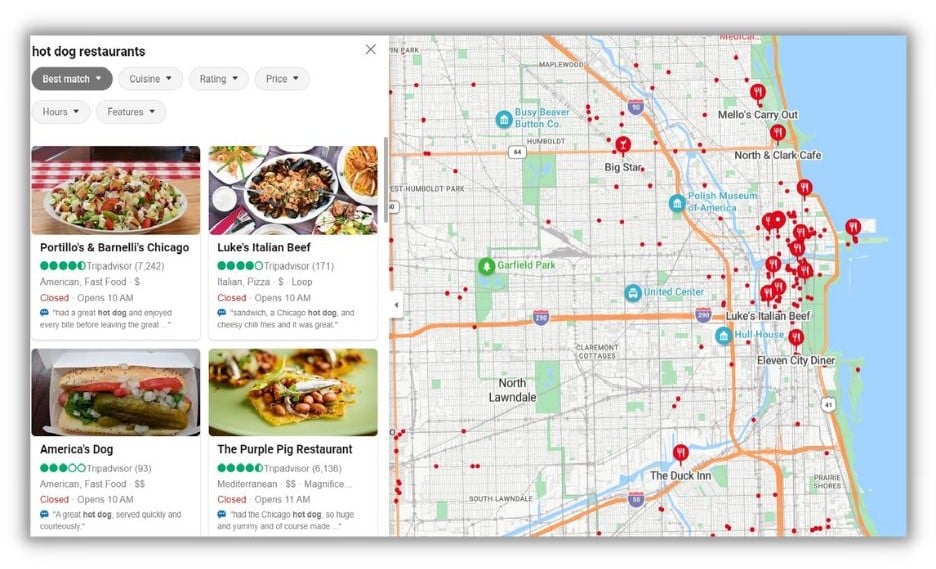The image showcases a detailed interactive map and restaurant search interface seamlessly integrated. 

On the right side of the image is a digital map peppered with red dots, resembling measles, pinpointing various locations. Notably, some pins cluster around a body of water, highlighting several restaurants each represented by a fork and knife icon, indicating their nature. 

To the left, a user appears to be searching specifically for hot dog restaurants. Below the search bar, results are filtered by "Best Match," and four prominent options are displayed:

1. **Portolinos and Barolinis, Chicago**: 
   - **Rating**: 4 out of 5 (as indicated by green dots)
   - **Cuisine**: American Fast Food
   - **Reviews**: 7200 reviews on TripAdvisor
   - **Details**: Includes opening hours, a brief review snippet, and a picture of their signature food item.

2. **Luke's Italian Beef**:
   - **Rating**: 4 out of 5 (green dots)
   - **Cuisine**: Italian, Pizza
   - **Price**: $ (affordable)
   - **Details**: Similar to above, it provides reviews, hours, and an image.

3. **American Dog**:
   - **Rating**: Not specified
   - **Cuisine**: American
   - **Price**: $$ (moderately priced)
   - **Description**: As before, reviews, operation times, and visuals are included.

4. **The Purple Pig**:
   - **Details**: Not fully elaborated but likely contains similar information as the top listings.

A route guidance feature akin to Google Maps is present, showing pathways to these eateries. Most of these restaurants are conveniently located near the Polish Museum of America, adjacent to the river, indicating a densely populated culinary hotspot.